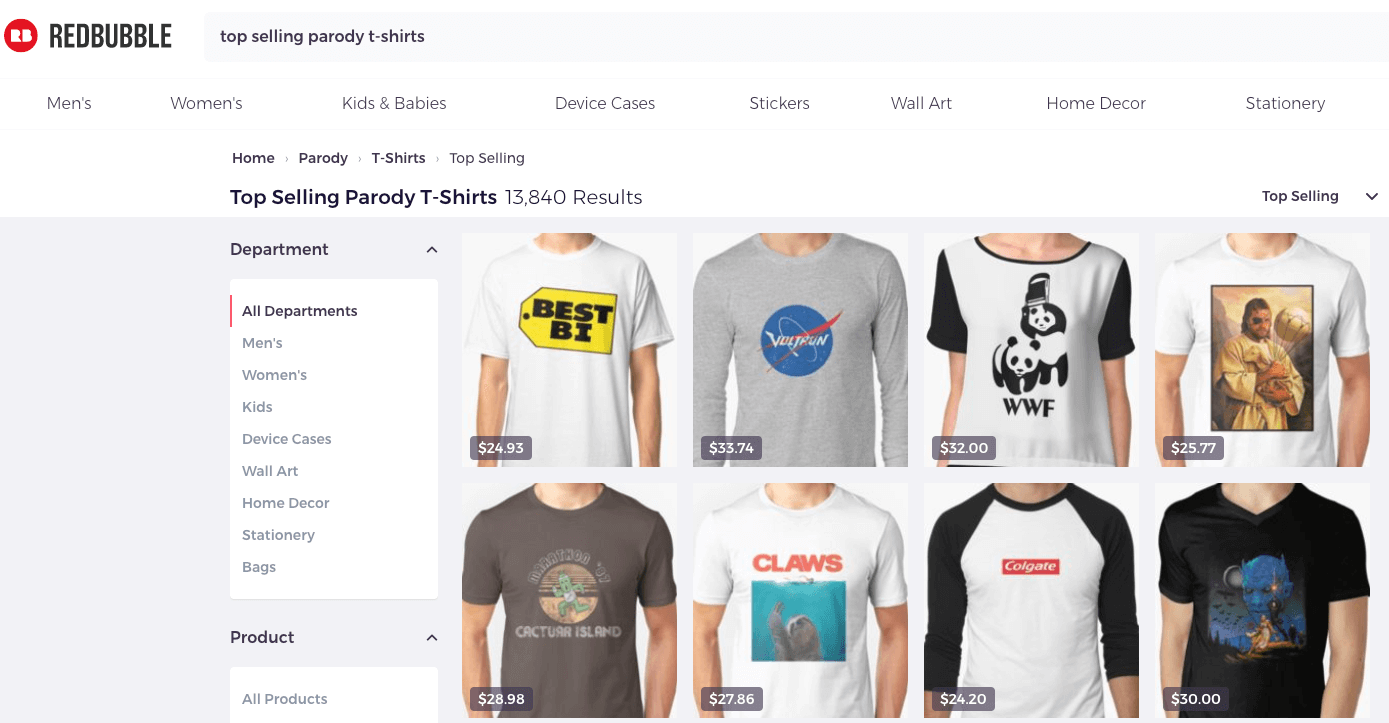The image is a horizontally rectangular screenshot from a retail website, specifically Redbubble. In the upper left corner, the website logo, "Redbubble," is displayed prominently. Directly across from the logo, there is a header that reads "Top-Selling Parody T-Shirts". Below this, a horizontal navigation menu lists various product categories: Men's, Women's, Kids & Babies, Device Cases, Stickers, Wall Art, Home Decor, and Stationery.

Beneath the navigation menu, the page header indicates that we are viewing the "Home" section for "Top-Selling Parody T-Shirts," displaying a total of 13,840 results. On the left side of the page, there is a vertical sidebar with a list of departments: All Departments, Men's, Women's, Kids, Device Cases, Wall Art, Home Decor, Stationery, and Bags. 

To the right of the sidebar, the main content area is organized into two rows, each containing four parody T-shirt images. For instance, the top-left T-shirt mimics the Best Buy logo, but the text inside the yellow price tag shape reads "Best Bi," with "Bi" spelled as B-I, instead of B-U-Y.